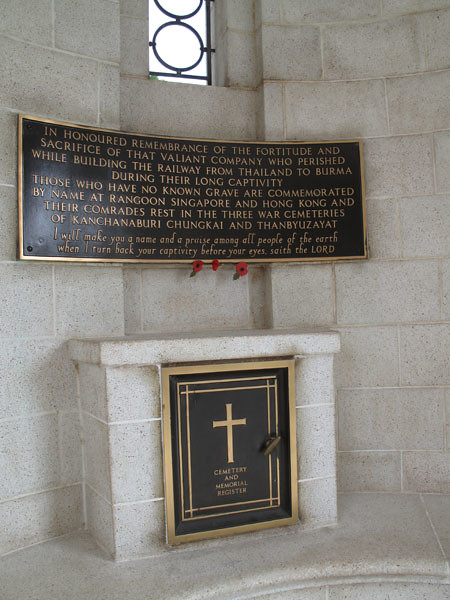The photograph captures a reverent section of a church, featuring a detailed memorial dedicated to those who perished while building the railway from Thailand to Burma. Central to the image is a large black plaque with gold trim, adorned with an inscription in gold lettering that reads, "In honored remembrance of the fortitude and sacrifice of that valiant company who perished while building the railway from Thailand to Burma during their long captivity. Those who have no known grave are commemorated by name at Rangoon, Singapore, and Hong Kong, and their comrades rest in the three war cemeteries of Ketchanaburi, Chiang Kai, and Thanh Bui Zayat." Above the plaque, a window with metal circles and black railing casts light onto the granite-colored stone wall. Below the plaque, red morning glory flowers add a touch of color, while a pedestal with a black plaque bearing a gold cross stands prominently. The bottom part of the memorial, resembling a concrete pedestal or fireplace, features the words "Cemetery and Memorial Register." A biblical verse inscribed on the plaque further honors the memory of the fallen, stating, "I will make you a name and a prayer among all people of the earth. When I turn back your captivity before your eyes, saith the Lord." The setting is solemn and respectful, creating a poignant tribute to the sacrifices made.